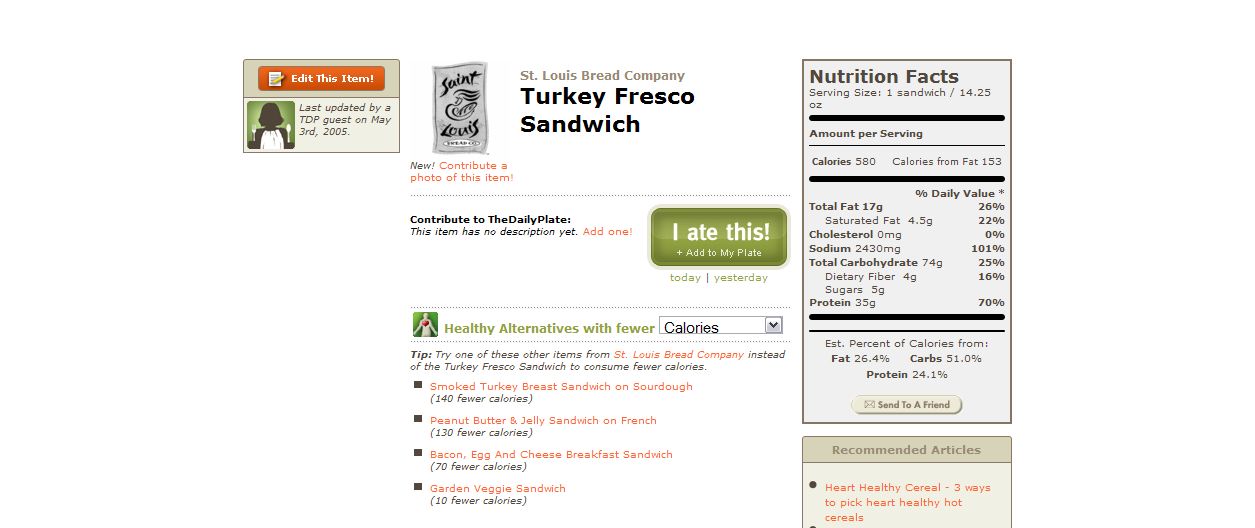This image is a digital screenshot from a website or app that provides detailed nutritional information for various foods. It's focused on the St. Louis Bread Company Turkey Fresco Sandwich. At the top, there's a small black and white company logo. To the left, a text box notes that the item was last updated by a TDP guest on May 3rd, 2005, with an orange button above it labeled "edit this item."

Centered on the page is the title "St. Louis Bread Company Turkey Fresco Sandwich" in prominent text. Below the title, an olive-green button marked "I ate this!" allows users to log the sandwich on their daily plate. Adjacent to this, a headline reads "Healthy alternatives with fewer calories," accompanied by a drop-down menu to explore other food options by calorie, carbohydrate, or fat content. 

On the right side, a comprehensive nutritional facts section lists the sandwich's ingredients and their corresponding percentages, grams, and weights. Below these details, there are links to similar sandwich options. This elaborate layout supports users in making informed dietary choices and contributing to the website's collaborative database.